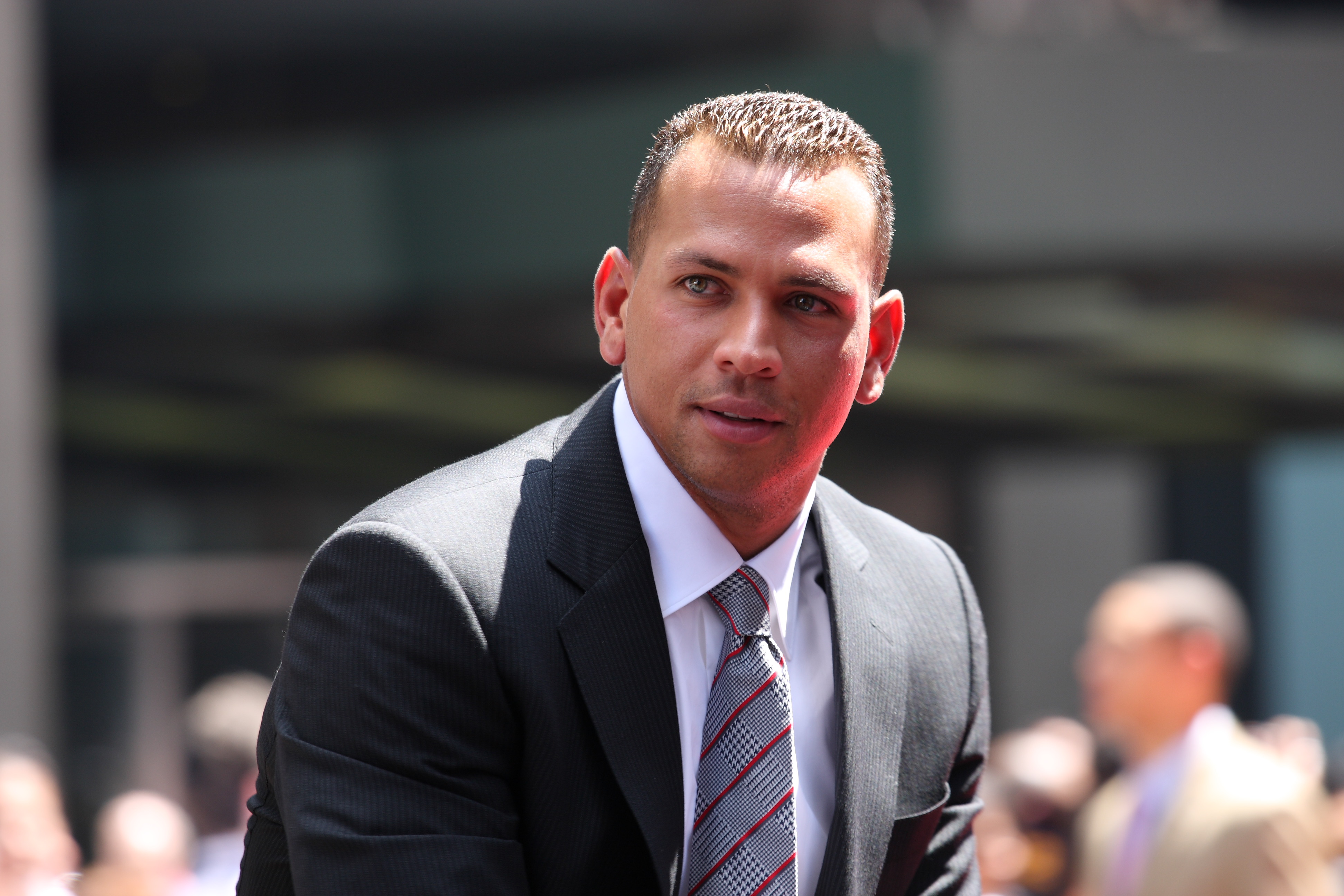The close-up photograph features a young, clean-cut Hispanic man, likely Alex Rodriguez. He has short, gelled brown hair combed to the front, slightly askew to his left. His sharp, crisp appearance is complemented by his attire: a dark gray pinstripe suit jacket that is left open, revealing a white button-down collared shirt and a distinctive gray tie. The tie features a mix of red diagonal stripes and subtle black and white designs. He seems to be in a good mood, with his mouth slightly open, and though his head is facing forward, his eyes gaze thoughtfully to the upper left. The background is blurred, hinting at some indiscernible structures and shapes of people, primarily in the lower corners, emphasizing the man's presence in the foreground. Only his torso, down to just above the elbows, is visible in this well-framed shot.